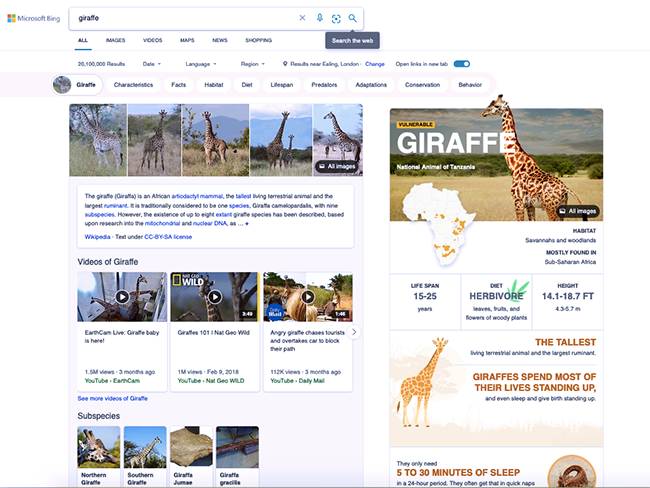A screenshot displays the results of a Microsoft Bing search for the term "giraffe" on a computer screen. The search results are categorized under various tabs such as All, Images, Videos, Maps, News, and Shopping, with the All tab currently selected. A search bar at the top includes a magnifying glass icon and text that says "Search the web." Below, it indicates the number of results found, the date, the language, and the region, including a clickable blue link labeled "Change" for adjustments. An option to open links in a new tab is activated, as shown by an on-position slider.

The results section prominently starts with the word "giraffe" and a thumbnail image of the animal. It includes subheadings like Characteristics, Facts, Habitat, Diet, Lifespan, Predators, Adaptations, Conservation, and Behavior. A variety of giraffe images populate the first row, displaying five different giraffe photos. Following this visual array is a detailed paragraph about giraffes. Below the introduction are three videos featuring giraffes, and further down, images of four subspecies of giraffes are shown.

On the right-hand side, a sidebar prominently features a large image of a giraffe along with extensive informational text, providing additional context and details about the species.